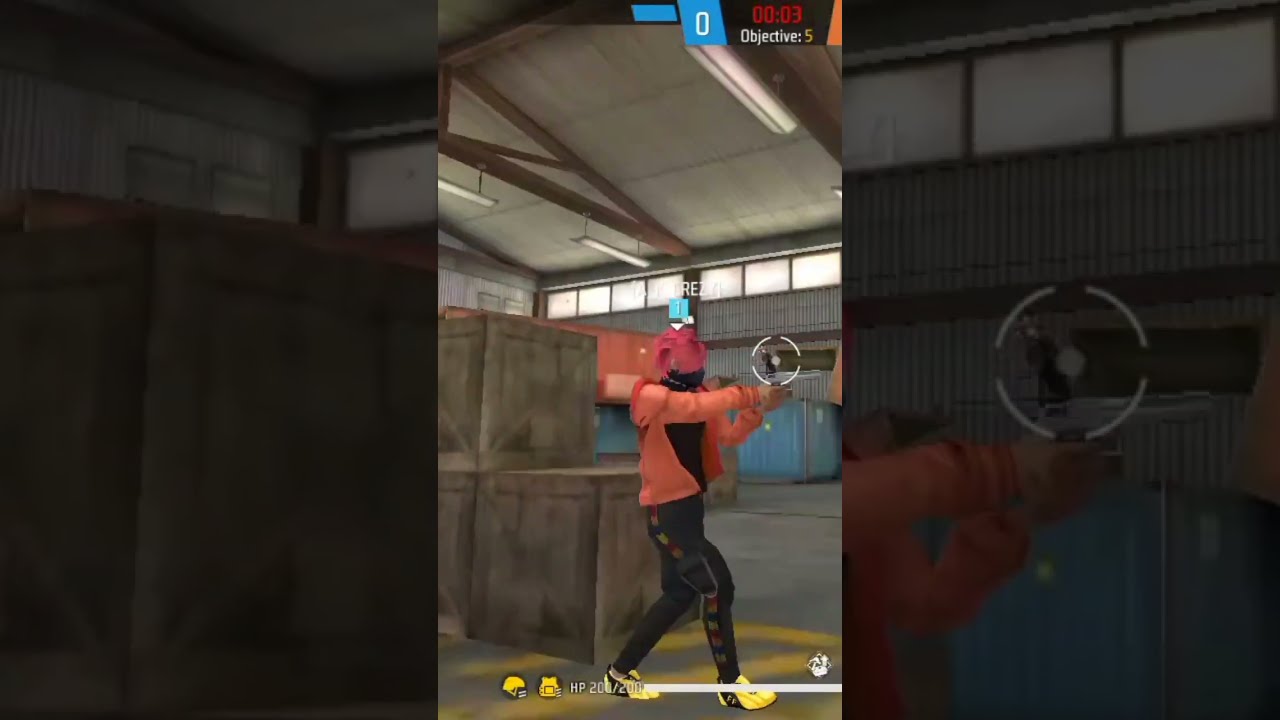In the center of a horizontally rectangular image, prominently featured in a clear vertical rectangle amidst a blurred surround, there's a dynamic scene that seems to be from a video game set inside a warehouse with metal rafters and gray walls. The left and right sides of the image are darkened, focusing the viewer's attention on the main action. In the foreground stands a character, identifiable by their bright attire and distinct stance. The character is wearing a soft orange long-sleeved hoodie over a black bodysuit, black pants adorned with colorful arrows, and yellow tennis shoes with black stripes. They have pink hair and a black mask that covers their face.

The character is depicted in an action pose, holding a large handgun with both arms extended, one arm higher and the other slightly lower, suggesting they are aiming or preparing to shoot. Their body is turned to the right, with one leg positioned forward as if in motion. Behind them, within the warehouse environment, are various elements like stacked square boxes and large blue containers, offering possible cover.

The game interface elements are visible, including a blue information square and a name tag above the character, and game statistics like “00.03 objective 5” on the top right. The bottom of the photo showcases items like a yellow helmet and a vest with "HP 200" indicated, hinting at the player's health status. This layered and detailed image captures the high-energy moment of gameplay within a distinctly industrial setting.